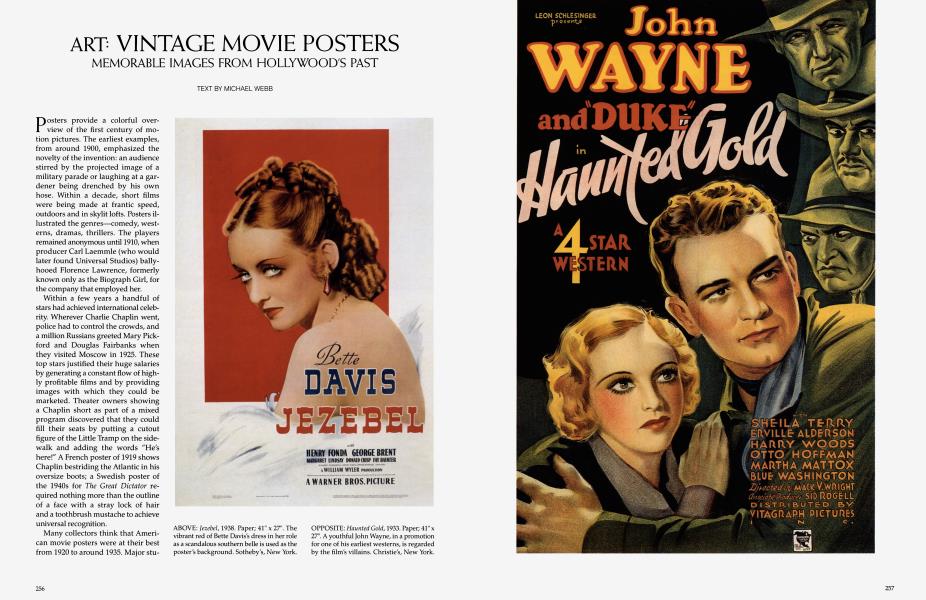The image depicts a two-page spread from an old magazine, featuring vintage movie posters and an article on Hollywood's past. On the left page, under a light gray background, the headline reads "Art, Vintage Movie Posters, Memorable Images from Hollywood's Past," with text by Michael Webb. There is a long, narrow column of text discussing early motion pictures and international celebrities. Beside the article, there is a stylized 1920s-esque illustration of Betty Davis for the movie "Jezebel," where she appears with thin eyebrows and dramatic makeup, her hair tied back in a low-hanging bun, seemingly topless but with shoulders and back visible. Beneath her image, it mentions "Warner Brothers Picture" and lists cast members.

On the right page, which appears to be a cover of a magazine or a featured movie poster, it showcases John Wayne and Duke in "Haunted Gold," a four-star Western. The poster displays a painting-like image of a fearful young couple in 1920s attire, the woman with a flapper hairstyle, embraced by a man in a dark green shirt, both looking off-camera. In the top right corner of the poster, there are three green-toned faces of men in old-time fedora hats, displaying expressions of anger or concern. The bottom right of the poster lists cast members, including Sheila Terry, Irville Alderson, Harry Woods, Ottoman Hoffman, Martha Maddox, Blue Washington, and directed by Mark Wright, in an orange font.